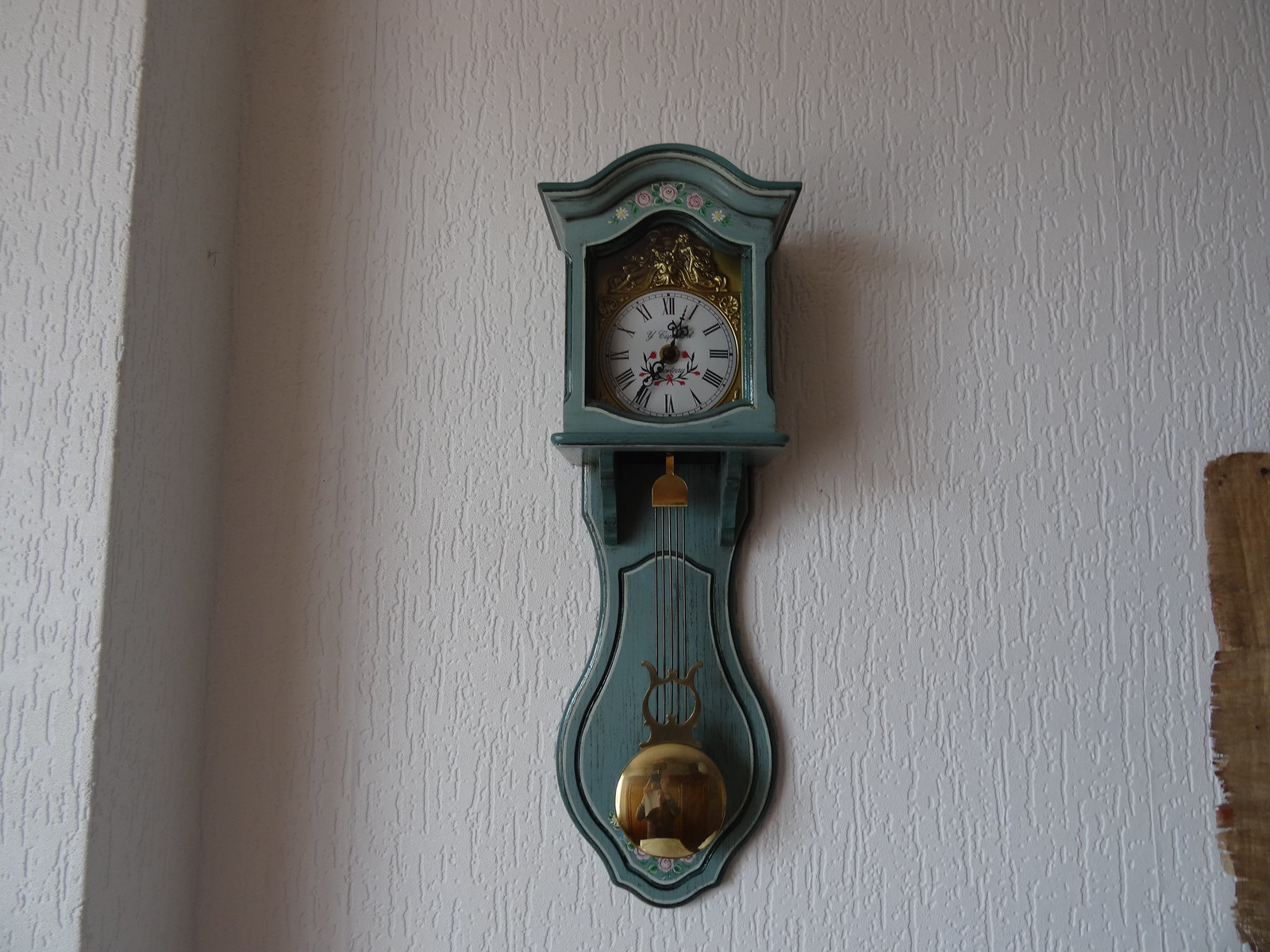This image showcases a vintage wind-up cuckoo clock, exuding a charming, old-school aesthetic. Crafted from wood and painted in a rich, dark teal hue, the clock embodies a nostalgic elegance. The time on the clock reads approximately 12:35. Its face is adorned with black Roman numerals and is encircled by a pure white background. Complementary black clock hands further accentuate the timeless design. Encircling the clock face are ornate gold embellishments, nestled within a scalloped top design that adds a touch of opulence. Extending from the bottom of the clock are strings that lead to a bell, indicative of the clock's traditional wind-up mechanism. The clock is mounted on a white, slightly textured wall, creating a striking contrast and highlighting its intricate details.